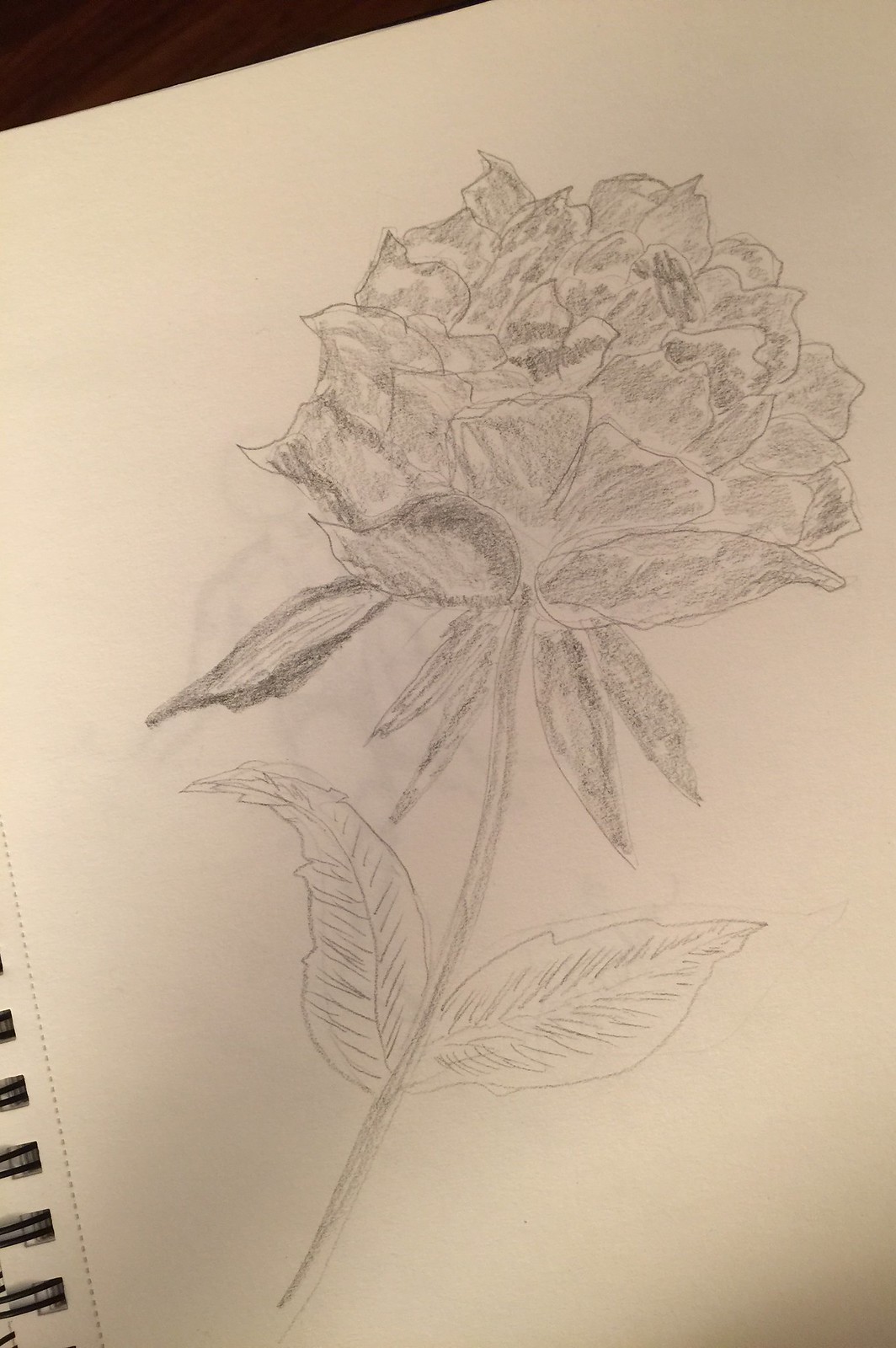This image showcases a detailed pencil sketch of a rose on a black spiral sketch notebook. The sketchbook is positioned at a sharp angle to the left, which accentuates the black spirals and perforated edges of the paper in the bottom left corner. In the top left corner, a glimpse of a dark wooden table is visible. The rose drawing features a long stem adorned with two large leaves; the left leaf extends outward to the left, while the right leaf points to the right. Both leaves display intricate pencil lines. The rose itself is rich in detail, with numerous petals intricately shaded with pencil. Notably, five petals at the base of the flower are angled downward, suggesting a wilting movement.